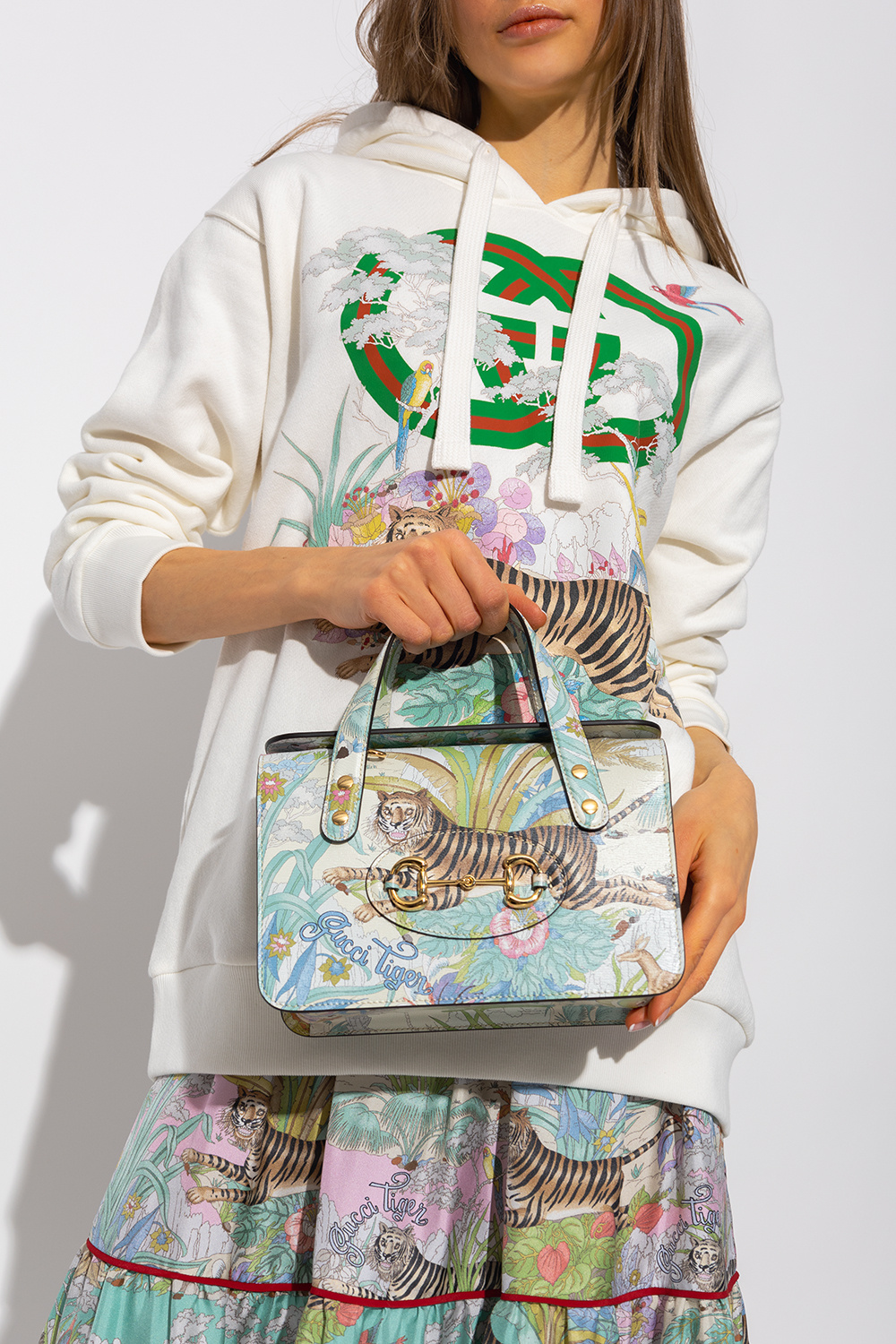This photograph showcases a young girl from the mouth down, with her dark straight, shoulder-length hair just visible. She is donning a coordinated outfit featuring a white sweatshirt with a distinctive green and red circular logo at the top, possibly resembling intersecting "G" and "C" letters, suggesting the Gucci brand. The sweatshirt prominently displays a cartoon tiger amidst vibrant flowers and plants, and a parrot, illustrating an enchanting scene. She holds a small, square lunch bag with two handles, akin to a clutch, featuring the same tiger image and the words "Gucci Tigers."

Her skirt complements the ensemble by depicting the same tiger scene, surrounded by an array of colorful flowers on a pastel background. The detailed, whimsical tiger motif extends across her entire outfit, blending into a cohesive and stylish look that emphasizes the brand's luxurious and distinctive design. The top section of the photograph is cut off, focusing the viewer’s attention on the playful and intricately designed attire.